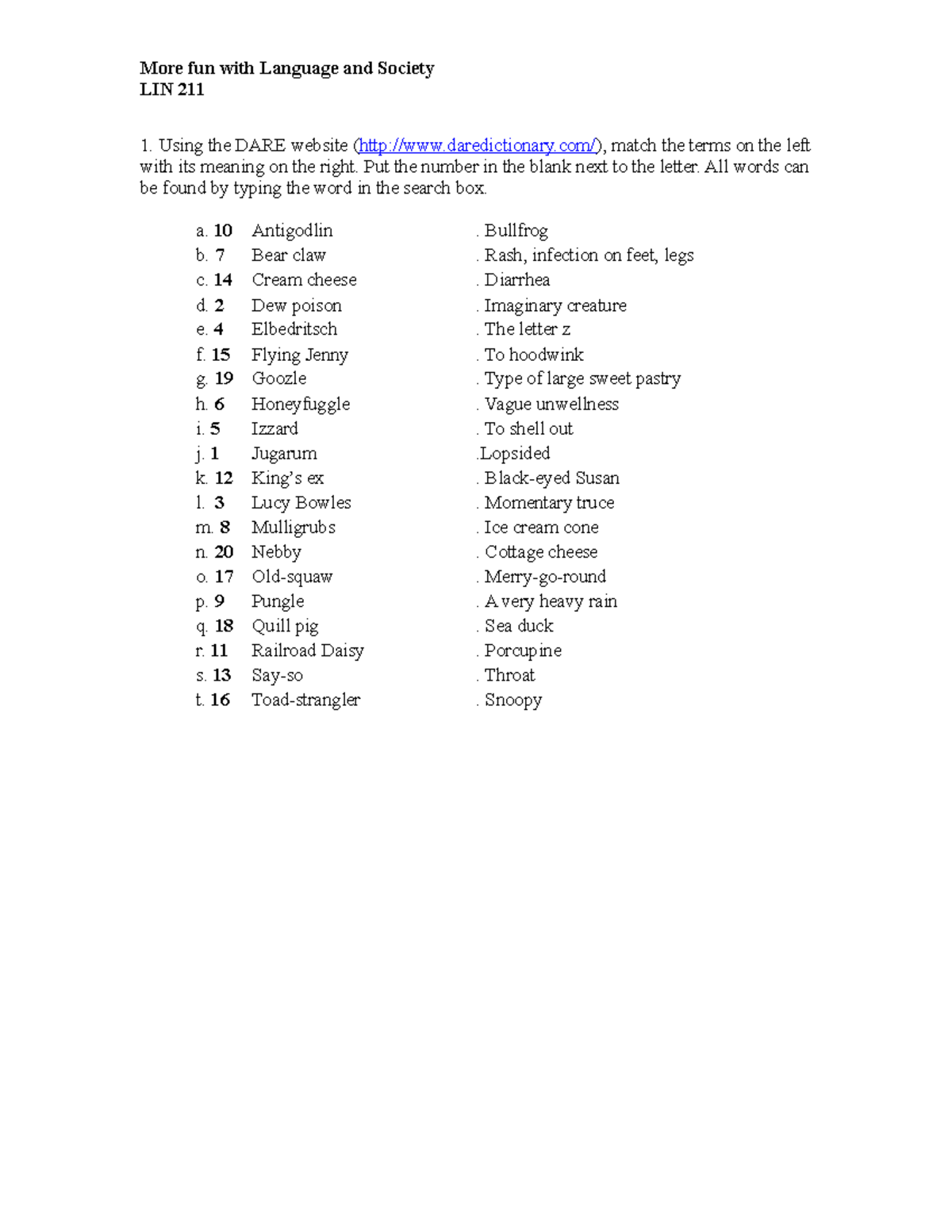The image displays an educational activity for LIN 211, titled "More Fun with Language and Society," prominently written in bold black letters at the top. It appears to be a game focused on language learning. The activity outlines the following instructions: "Using the D.A.R.E. website (http://www.daredictionary.com), match the terms on the left with their meanings on the right by putting the corresponding number in the blank next to the letter. All words can be found by typing them in the search box."

The left side of the image lists terms paired with bolded numbers:

- A. 10 Antigodlin
- B. 7 Barakal
- C. 14 Cream Cheese
- D. 2 Dew Poison
- E. 4 Albedritch
- F. 15 Flying Jenny
- G. 19 Goozle
- H. 6 (blank)
- I. 5 Izzard
- J. 1 Jugaroom
- K. 12 King's X
- L. 3 Lucy Bowles
- M. 8 Molly Grubbs
- N. 20 Nabby
- O. 17 Old Squaw
- P. 9 Pungle
- Q. 18 Quail Pig
- R. 11 Railroad Daisy
- S. 13 Say-So
- T. 16 Toad Strangler

On the right-hand side, a bulleted list of definitions is provided:

- Bullfrog
- Rash
- Infection on Feet
- Legs
- Diarrhea
- Imaginary Creature
- The letter Z
- To Hoodwink
- Type of Large Sweet Pastry
- Vague Unwellness
- To Shell Out
- Lopsided
- Black-Eyed Susan
- Momentary Truce
- Ice Cream Cone
- Cottage Cheese
- Marigold Round
- A Very Heavy Rain
- Sea Duck
- Porcupine
- Throat
- Snoopy

Participants are required to use the D.A.R.E. website to find the meanings of the terms and correctly match the numbers to their definitions.